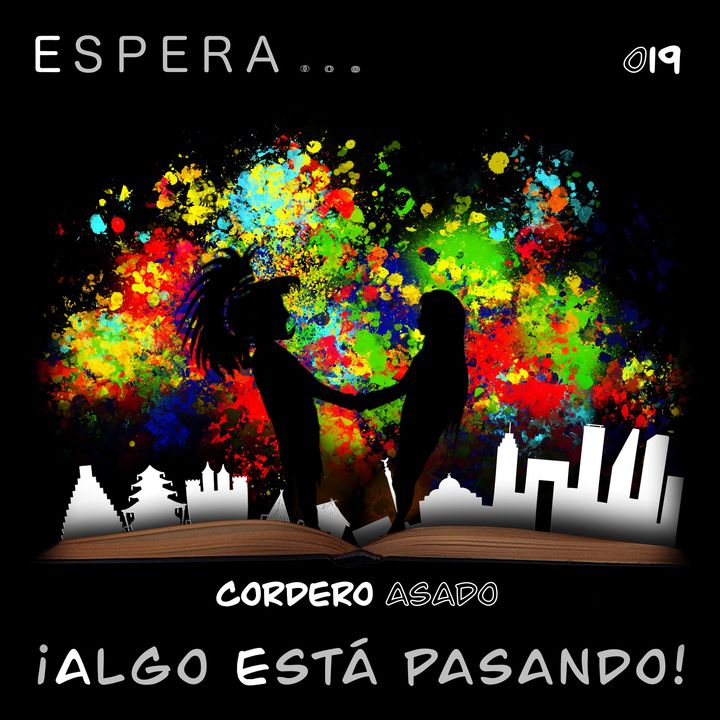The image, rendered in either a drawn or computer graphic style, features a striking black background. At the center, a vibrant splatter of colors—red, yellow, green, turquoise, and dark blue—bursts forth, reminiscent of a paintball impact. This dynamic backdrop frames the silhouettes of two people shown in profile, standing and holding hands. The person on the left sports a high ponytail and possibly a goatee, while the person on the right appears to be wearing a large headdress, characterized by long hair or elaborate adornment. These figures stand in front of the outlined silhouettes of various buildings, depicted in white and resting on the outline of an open book.

Text is strategically placed across the image. At the top left, the word "ESPERA" is displayed, with the letter "E" in white and the remaining letters in gray. The top right corner features the digits "019," with the first digit in black outlined in white, and the remaining digits in white. At the bottom of the image, the phrase "CORDERO ASADO" is prominently situated, with "CORDERO" in white and "ASADO" in black with a white outline. Directly beneath this, the statement "ALGO ESTA PASANDO" appears in white text.

The entire composition combines elements of street art aesthetics with abstract, vivid colors and symbolic silhouettes, enriched by textual components that add a layer of intrigue and context.